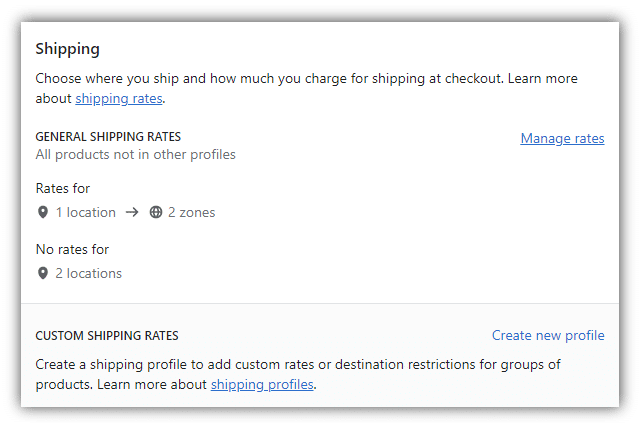This image is a detailed visual representation of a shipping information dashboard with a white background and predominantly black text. 

- At the top left corner, the heading "Shipping" is prominently displayed.
- Below the heading, there's a descriptive line: "Choose where you ship and how much you charge for shipping at checkout."
- A blue, clickable link labeled "Learn more about shipping rates" is available.
- The section "General Shipping Rates" follows, noted as applicable to all products not assigned to other profiles.
- To the right of this section, the phrase "Manage rates" is underlined in blue, indicating another clickable link.
- On the left side, a subsection titled "Rates for" features icons: a pin icon next to "One location" and a globe icon next to "Two zones."
- Below, it states "No rates for" followed by a pin icon next to "Two locations."
- At the bottom, in capital letters, the text "Custom Shipping Rates" stands out.
- Underneath, it instructs users to "Create a shipping profile to add custom rates or destination restrictions for groups of products."
- Another blue, underlined link labeled "Shipping profiles" invites users to learn more.
- On the right side, there's a prominent button labeled "Create new profile."

This comprehensive layout provides clear instructions and interactive elements for managing shipping rates.